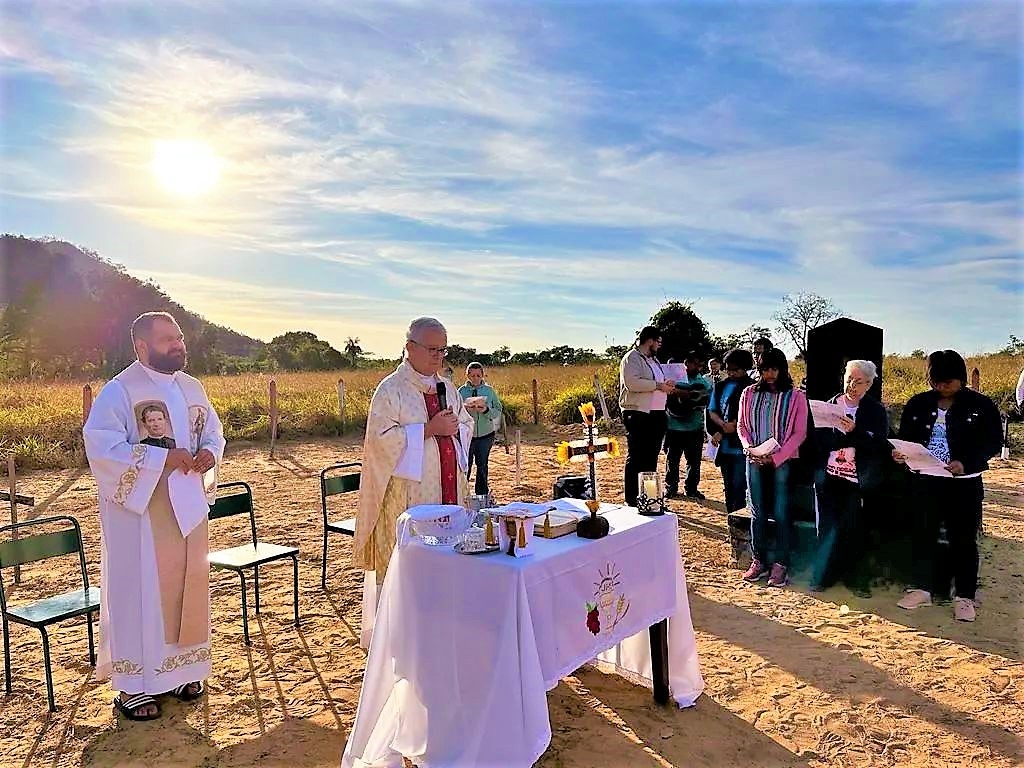In a full-color, square photograph taken outdoors on a partly sunny day, a peculiar religious gathering is captured. The image shows a dirt clearing set within a larger grassy field, bordered by wooden stakes and flanked by trees and tall grass. The top half of the image is dominated by the sky, with clouds partially obscuring the sun on the left side, and a wooded hill can be seen in the center-left background.

In the lower half of the image, a group of 10 to 15 people are assembled. Dominating the scene is a table draped with a white tablecloth positioned centrally, with various items on it, including a bowl and an upright cross. Behind this table stands a man in flowing beige and red religious garb, speaking into a microphone, seemingly leading the ceremony. To his left is another man also in religious attire, though slightly different, adorned with a picture of a man on his right breast and notably wearing black Adidas sandals with white stripes.

Most people in the crowd wear a mix of semi-formal and casual attire, with a few dressed in black, possibly suggesting a somber occasion such as a funeral. Some attendees are holding booklets or folders, likely reading from them, contributing to the atmosphere of a communal ritual. The stark contrast between the pale dirt ground and the vibrant greenery around them, combined with the diverse attire of the participants, adds to the enigma of this outdoor religious event.